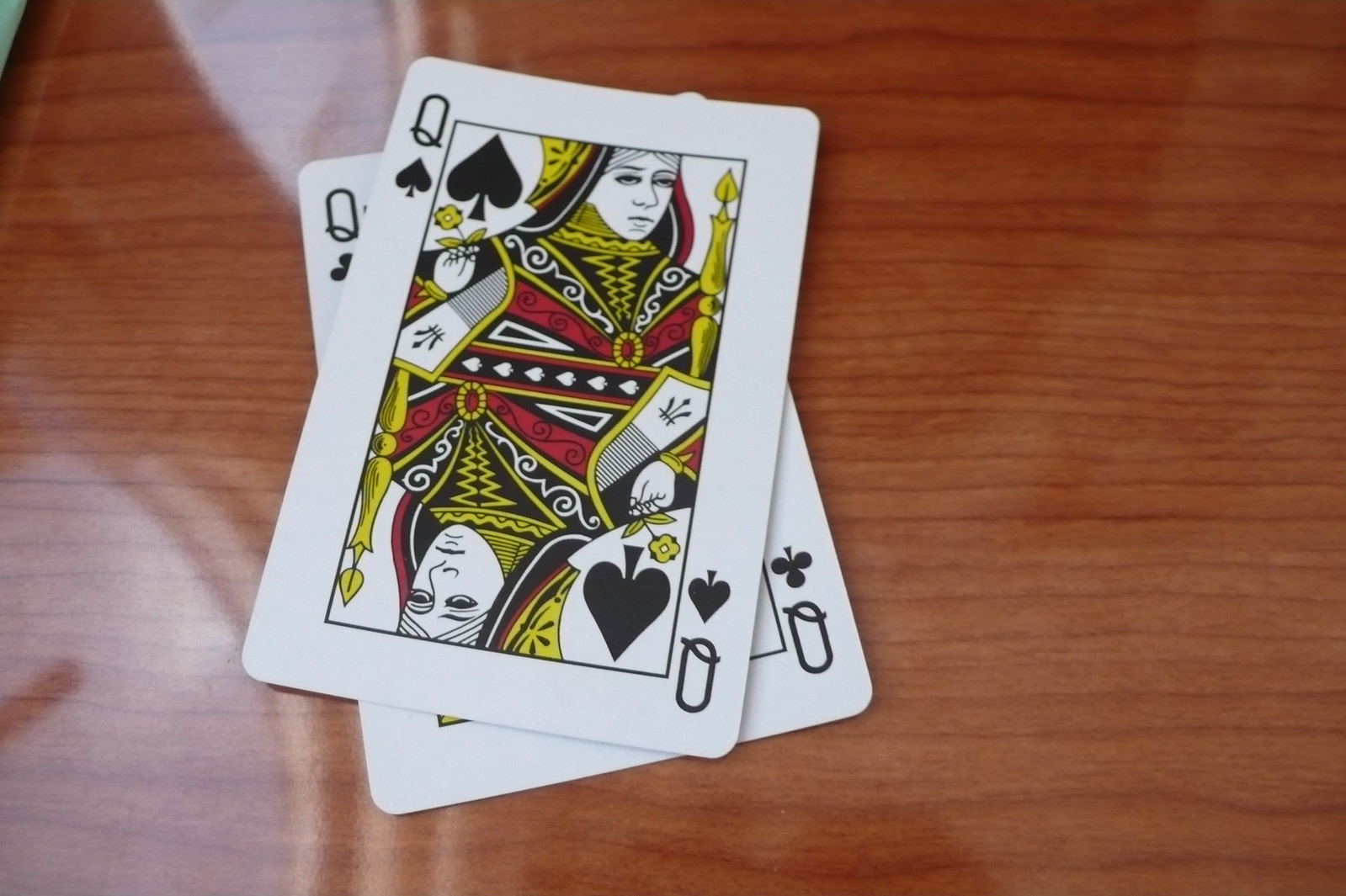This photograph features a table, possibly a coffee or kitchen table, with a light brown surface accented by horizontal darker brown streaks. On this table, there are two playing cards: the Queen of Spades on top and the Queen of Clubs beneath it, both in black suits. A shadow casting the shape of a cup with a straw is visible in the bottom left corner. Additionally, there's a glare in the top left of the image that appears blurred, rendering its source indiscernible. The very top left corner of the photograph shows a small white object, possibly a plate or a cup, which is also not clearly identifiable.